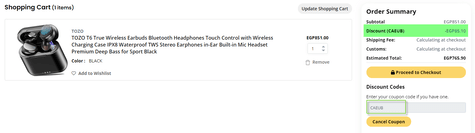This screenshot captures a small section of a shopping cart interface. At the top, it indicates that there is "1 item" in the cart. To the right, there's a prominent gray button labeled "Update Shopping Cart." Below that, the product details are listed: "TOZO T6 True Wireless Earbuds Bluetooth Headphones," featuring touch control, a wireless charging case, waterproof TWS stereo earphones, in-ear design, and a built-in mic, all boasting premium deep bass, ideal for sports. The color specified is black. An "Add to Wishlist" button lies beneath this description.

Adjacent to these details, there's a quantity selector box displaying the number "1," with arrows to increase or decrease the quantity. Below this, a trash can icon offers the option to remove the item from the cart. On the far left, a high-resolution image showcases the product: a sleek and glossy black box with a lift-up lid, revealing the two earbuds neatly nestled inside.